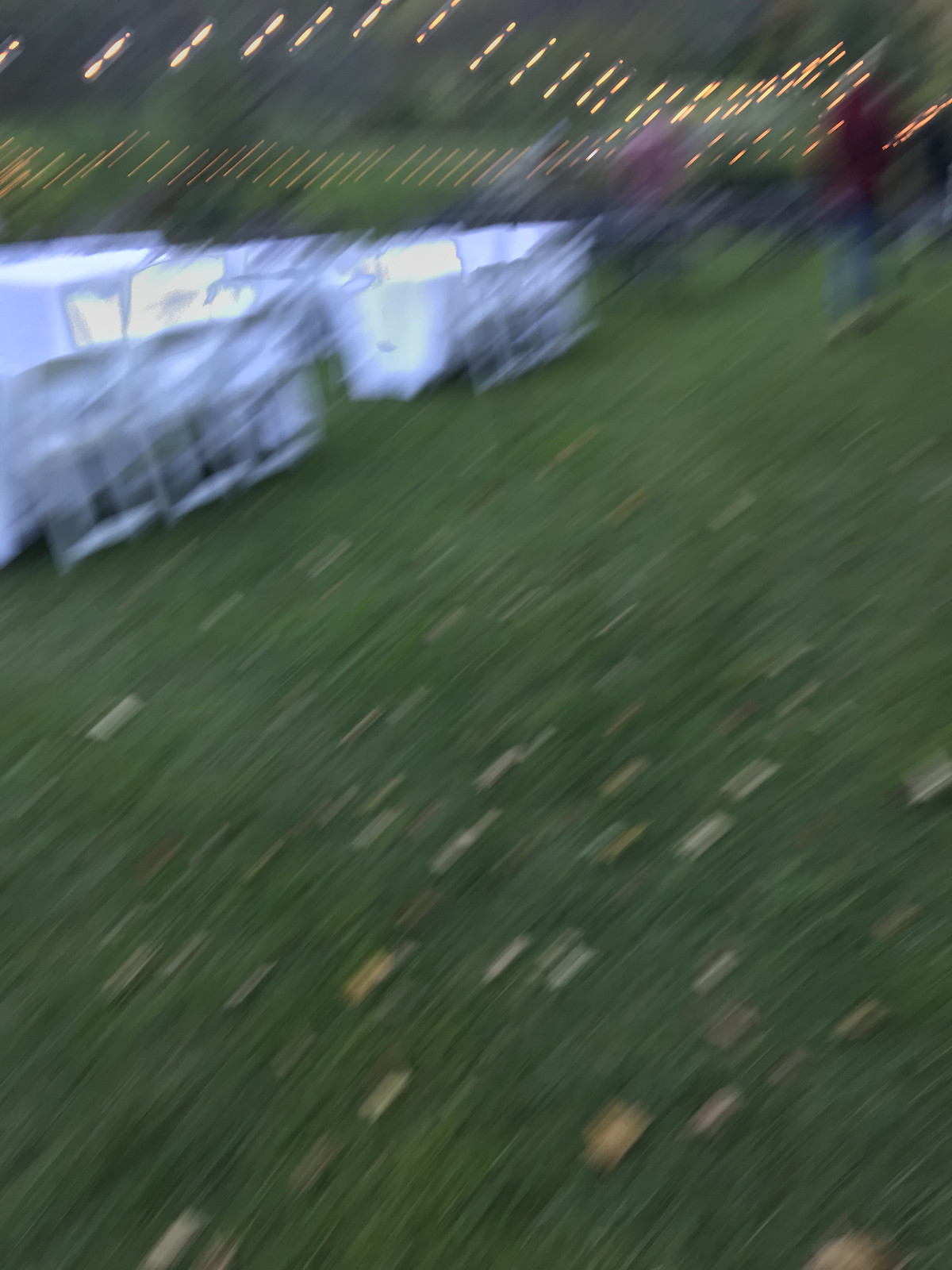A blurry outdoor photograph captures a scene with various elements. The upper portion of the image features strings of lights extending from the left to the right. Below, there is a setup of white chairs around a table draped with a white tablecloth. In the top right corner, a person dressed in a maroon shirt and jeans stands amidst a group of people. The majority of the lower half of the photo shows a grassy area scattered with square objects in yellow and white.